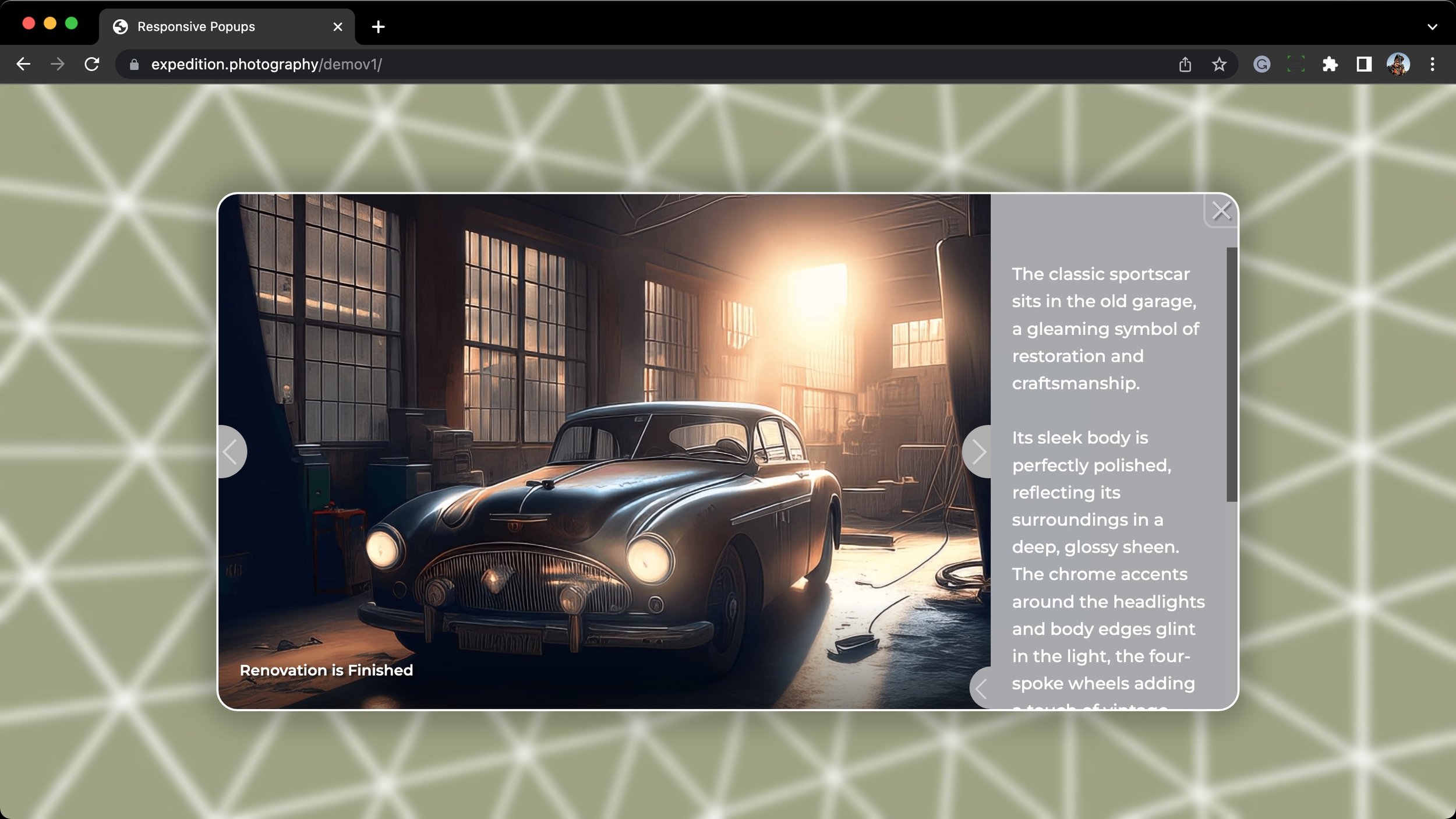The image depicts the desktop of a Macintosh computer with the familiar three small circles—the red, orange, and green dots—in the top left corner, indicative of a Mac interface. The browser displayed is Google Chrome, with the open tab labeled "responsive pop-ups." The address bar shows the URL "expedition.photography/.demo v1/" along with icons for bookmarks, upload, and the user's profile with quick access to their apps.

The central focus of the webpage is a classic 1950s-style sports car showcased in an old garage, bathed in sunlight streaming through the windows on the left side. The garage’s atmosphere is further highlighted by the presence of various tools scattered on the floor. The car is immaculately restored, with its sleek, polished body reflecting the surroundings in a deep, glossy sheen. Chrome accents around the headlights and body edges glint under the light, adding a touch of elegance. The partially visible text alongside the image reads: "The classic sports car sits in the old garage, a gleaming symbol of restoration and craftsmanship. Its sleek body is perfectly polished, reflecting its surroundings in a deep, glossy sheen. The chrome accents around the headlights and body edges glint in the light. The four-spoke wheels…" implying further detailed description trails off. At the bottom left corner of the image, the text "Renovation is finished" can be seen, concluding the visual narrative of this impeccably restored vehicle. 

In the background, the webpage design features an olive triangular pattern with white borders, adding an aesthetic geometric touch to the overall presentation.